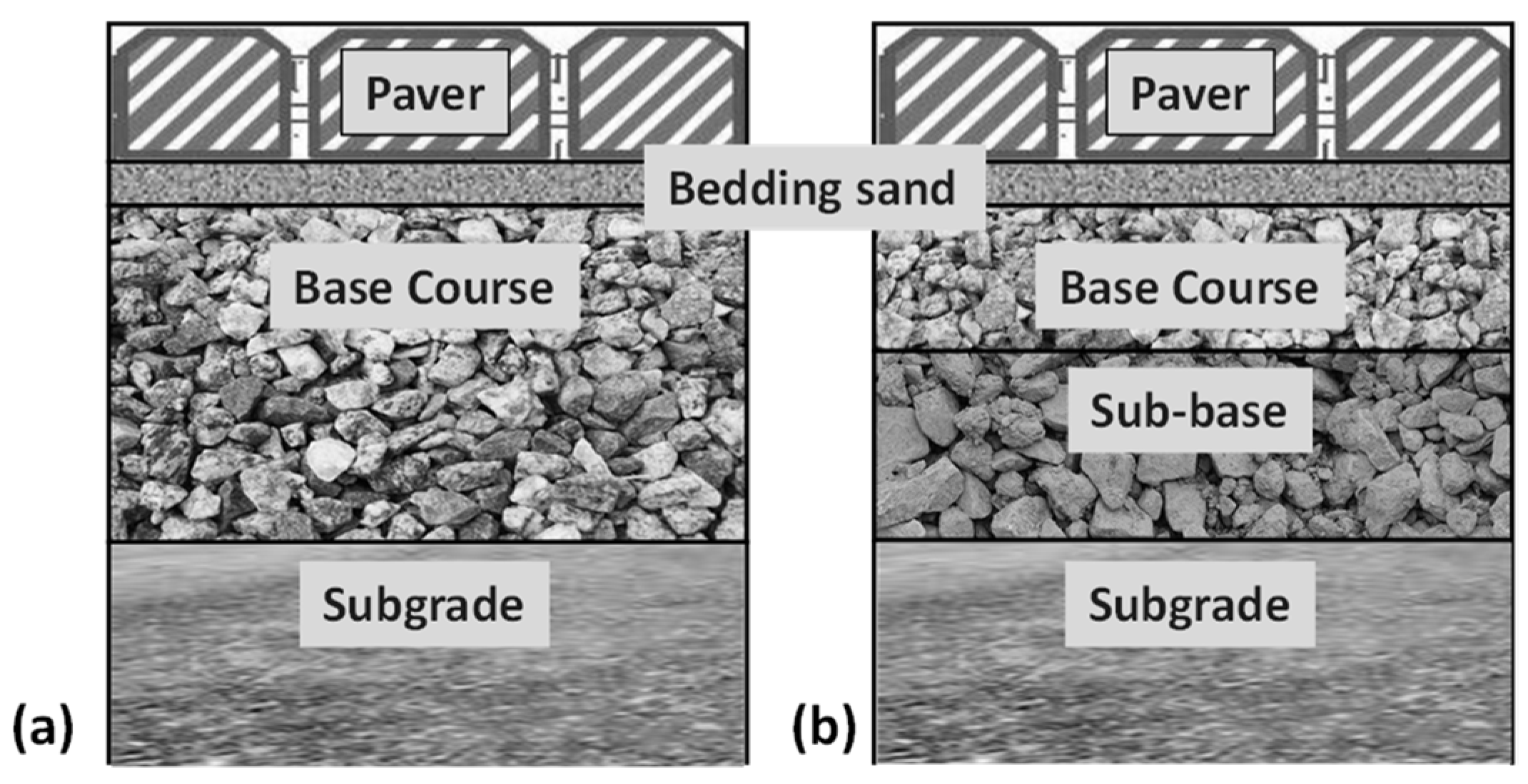The diagram is a black and white illustration, likely meant to show the structure of a road or similar construction. It features two side-by-side sections labeled 'A' on the left and 'B' on the right. Both sections display layered materials, with some key differences.

In both sections, the bottommost layer is labeled 'subgrade,' depicting the foundational ground layer. Moving upward, Section A shows a single intermediate layer labeled 'base course,' represented by large gravel. Above this is a narrow strip labeled 'bedding sand,' and the topmost layer is marked 'paver,' featuring bricks with stripes and a sign in light blue with dark blue lettering saying "paver".

Section B, on the other hand, has two intermediate layers between the 'subgrade' and the 'bedding sand.' Directly above the 'subgrade' in B is a layer labeled 'subbase,' consisting of large gravel, and above that is another layer marked 'base course,' also large gravel. Similarly, a narrow 'bedding sand' layer sits above these, topped by the 'paver' layer identical to that in Section A.

The two sections are side-by-side with a white space between them, presenting a clear visual comparison between the single 'base course' layer in Section A and the additional 'subbase' layer in Section B.